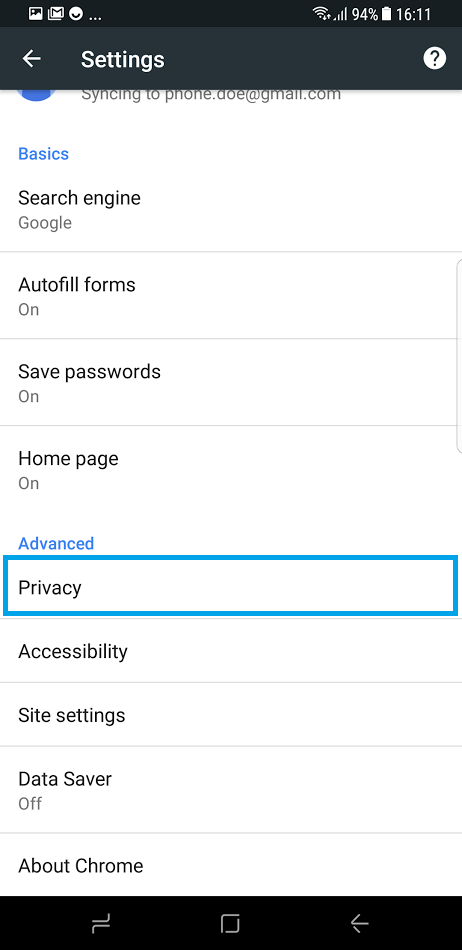This image is a screenshot taken from the settings menu on a smartphone. At the very top, there's a black rectangular notification bar featuring various icons. On the left side of the bar, there are unidentified icons, while the right side displays indicators for battery life (showing 94%), Wi-Fi connection, and signal bars. The current time is also visible, shown as 16:11.

Just below the notification bar, there's a header section with the word 'Settings' prominently displayed in white. Accompanying this is a left-pointing arrow on the left side. On the far right side of this header section, a black question mark inside a white circle is visible. Partially cut off at the very top of the settings menu, there's a statement indicating that the phone is syncing to an email address (highlighted as phone.doe@gmail.com), next to which a blocked profile picture is faintly visible.

Below this header, the settings menu displays the section title 'Basics' in blue, indicating it is clickable. Following this, several settings options are listed: 'Search engine,' which is set to 'Google,' and 'Autofill forms,' showing the status 'On' in gray text. Each of these options is separated by faint gray dividers.

Further down, 'Save passwords' is another setting listed as 'On,' followed by another faint gray divider, and 'Home page,' which is also turned 'On.' At the bottom of the visible settings list, there are clickable options labeled 'Advanced' and 'Privacy' in blue. This entire section is bordered by a thin teal line forming a rectangle around it.

Overall, this detailed screenshot shows various customization options within the settings menu, highlighting important aspects such as connectivity status, account syncing, and various operational settings.